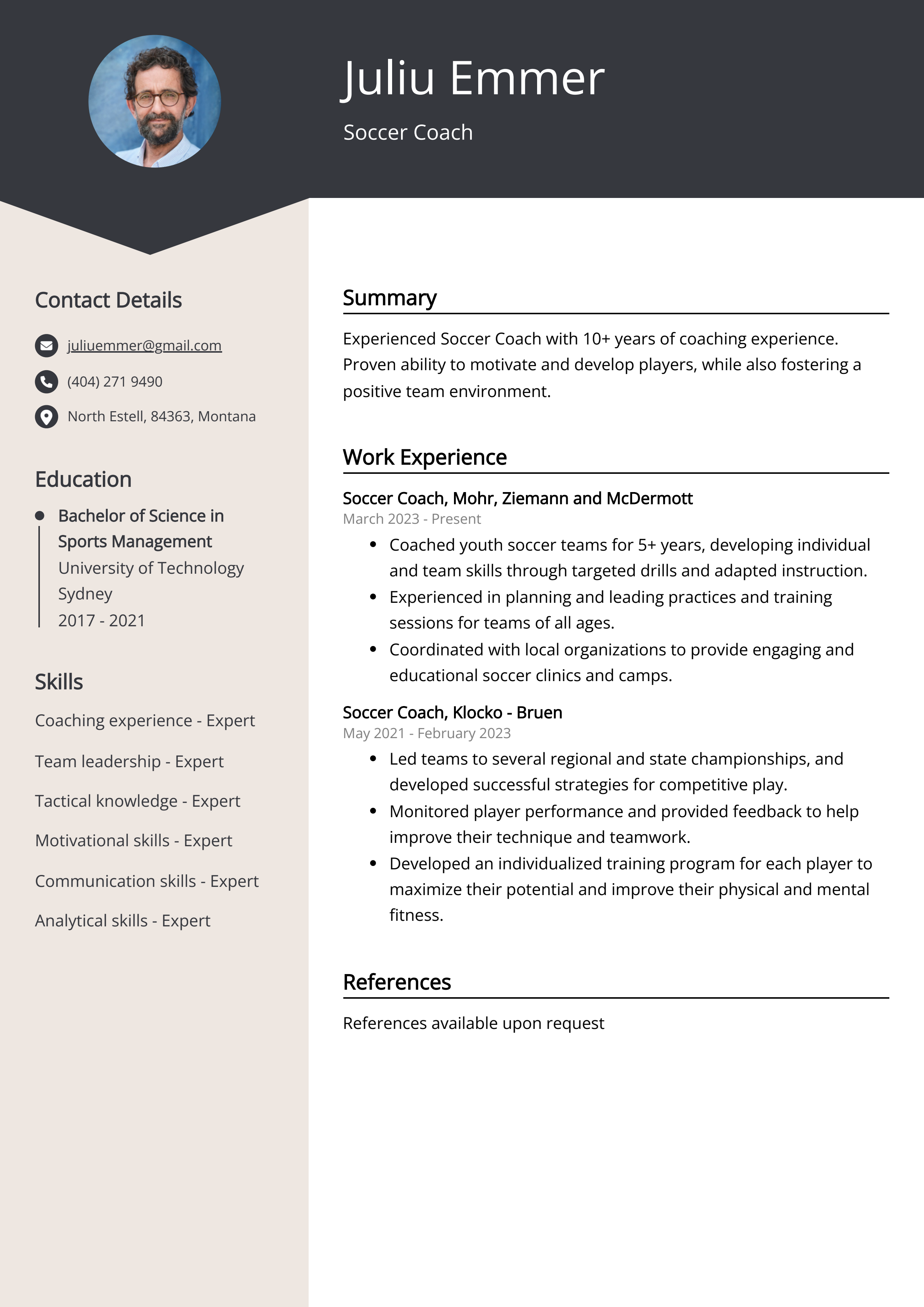This image portrays the detailed resume of Juliu Emmer, a seasoned soccer coach. At the top, against a black background, the name "Juliu Emmer" is prominently displayed. A headshot to the left features Juliu wearing glasses, a collared shirt, and sporting short brown hair, a beard, or goatee, set against a blue background. The left column, accentuated by a light grayish-brown rectangle, lists his contact details, residence, and educational background, specifically a Bachelor of Science in Sports Management. His skills listed include coaching experience, team leadership, tactical knowledge, motivational and communication skills, and analytical proficiency, with an expert level of competency claimed across these areas.

The right section features a white background that holds a summary of Juliu's career, highlighting his decade-long experience in coaching. He has worked as a soccer coach at Moore, Zeeman, and McDermott, as well as at Klucker Bruin. Contact details, detailed work experience, and references (available upon request) are all neatly organized within this section, offering a comprehensive view of Juliu Emmer's professional qualifications and background.